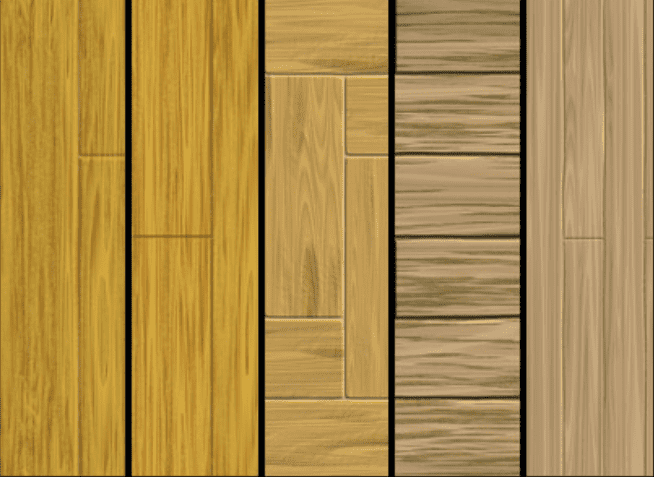This image showcases a sample sheet of wooden panels, likely displayed in a hardware store such as Home Depot or Lowe's. The display comprises five distinct vertical columns of wood panels, each separated by thin black lines. From left to right, the panels exhibit a variety of wood grains and colors.

The first panel on the left is vertical with a brighter yellow hue. The wood grain runs vertically. The second panel, also vertically aligned, has darker brown shades interspersed within its grain. The third, central panel is uniquely patterned with both vertical and horizontal wood grains and is divided into a series of geometric sections: a square at the top, a central vertical rectangle adjacent to a smaller square on the right, a long skinny vertical rectangle, and a square beneath it. The fourth panel stands out with a dark brown hue and horizontal wood grain. Finally, the panel on the far right is light tan with vertical wood grain featuring a lighter tint and some white streaks. These details suggest a diverse selection of wood flooring samples designed to illustrate the variety available for different home applications.